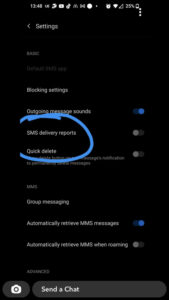**Detailed Caption:**

A blurred screenshot of a smartphone settings menu with a black background and white text. Highlighted by a blue circle is the "SMS Delivery Reports" option, which is currently turned off. The screenshot is slightly blurry, making some of the text hard to read. At the top of the screen, there are various status icons including YouTube, clock, Wi-Fi, battery at 25%, and a timestamp that is unclear. Below these icons, a left-facing arrow labeled "Settings" is shown. Further down, there are various settings options listed.

One partially readable section mentions "Outgoing message sounds," with its toggle button switched on. Following this, the highlighted "SMS Delivery Reports" option is visible. Another setting, possibly related to "Quick responses," is indicated but also turned off. Below these, there is a section possibly referring to "MMS Group Messaging," with a setting to "Automatically receive MMS messages" turned on, and another option for "MMS while roaming" turned off.

At the very bottom of the screenshot, a camera icon and a text box for sending a chat are visible.